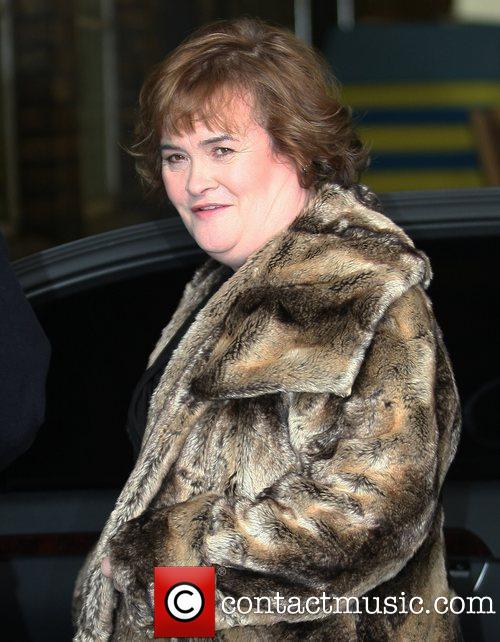The image features Susan Boyle in a side view, capturing her left profile. She appears to be in her late 50s to early 60s and is dressed in a luxurious fur coat with shades of beige, light brown, and dark brown, interspersed with black and gray. Her short, wavy auburn hair falls just below her ears, and she has a slight smile on her face. Susan is positioned centrally in the frame, looking off slightly to the right. The background is very dark and blurry, but it hints at an outdoor environment with some indistinct yellow horizontal lines in the upper right. Behind her is a vehicle, partially visible with dark windows and a dark paint job. The lower right corner of the image features a small red square with a black circled "C," accompanied by the text "contactmusic.com" in white.